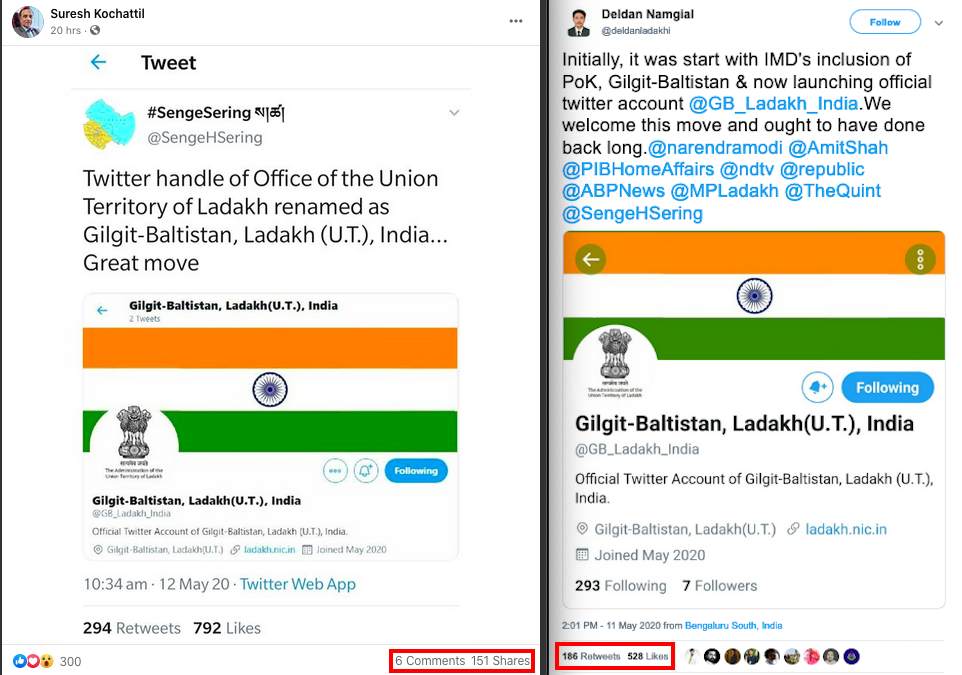The image consists of two tweets related to the social media platform Twitter. The tweets detail updates from official accounts about geopolitical changes.

**Left Image:**
- **Username:** Suresh Kachadal
- **Timestamp:** 20 hours ago
- **Tweet Content:** 
  - The tweet includes the hashtag #SingeSyringe, along with some text in another language.
  - It mentions the official Twitter handle of the "Office of the Union Territory of Sadaq," which has been renamed to Gilgit-Baltistan Ladakh (UT India).
  - **Tweet Text:** "Great move."
  - **Attached Image:** A flag featuring orange and green colors with a blue circle in the center.
  - **Metrics:** The tweet was posted at 10:34 AM on May 12, 2020, from the Twitter web app. It has received 294 retweets and 792 likes.

**Right Image:**
- **Username:** Delden Namgyal
- **Twitter Handle:** @DeldenLadakhLadakhi
- **Follow Button:** Present to indicate the option to follow the user.
- **Tweet Content:**
  - The tweet discusses the inclusion of POC Gilgit-Baltistan by the Indian Meteorological Department (IMD) and the launch of the official Twitter account @GBLadakhIndia.
  - **Tweet Text:** "Initially it started with IMD's inclusion of POC Gilgit-Baltistan, and now launching official Twitter account @GBLadakhIndia. We welcome this move; it should have been done long ago."
  - **Attached Image:** The same flag is shown, representing the discussed region.
  - The tweet includes several mentions of other Twitter handles highlighted in blue.

The text has been cleaned up to clearly portray the nature of the tweets, emphasizing their content, timestamps, metrics, and attached images.